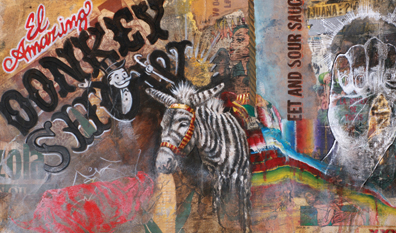The image is an intricate and colorful mural-style painting, displaying a diverse mix of vibrant artwork with elements of both abstraction and surrealism. Central to the image, a donkey-like figure with black stripes and an orange-red halter stands prominently, adding a striking feature to the composition. At the top left corner, red cursive text spells out "L. Amazing," just above bold, black text declaring "Donkey Show." Below the donkey, a man with a pockmarked face and large red lips can be seen, enhancing the mural’s eclectic feel.

On the left side of the image, amidst the myriad of colors, a red smear is encircled by white smoke, adding texture and visual intrigue. Beneath "Donkey Show," the iconic Monopoly Man emerges from the "O" with his signature top hat, cane, and handlebar mustache, blending seamlessly into the chaotic and colorful backdrop. He appears delighted, contributing a touch of whimsy and humor to the painting.

Toward the right, the mural showcases a large, faintly visible white fist, juxtaposed against a graffiti-like pattern featuring shades of blue, red, and green, possibly on a building facade. Scattered among these visuals are segments of foreign text that enhance the mural’s mystique. Adding another layer of quirkiness, the words "Sweet and Sour Sauce" are discernable, climbing up the image, interweaving with the overall abstract and vibrant theme of the artwork.